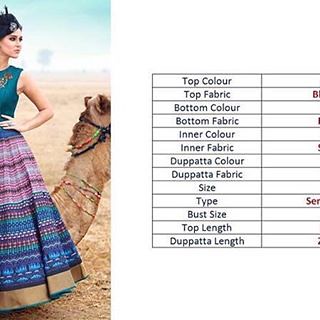The image showcases a photorealistic drawing of a light-skinned woman with her black hair done up, wearing an elaborate sleeveless turquoise blouse and a flowing skirt adorned with intricate patterns in blues, purples, whites, and tans. She stands with her left hand on her waist, a large ring on her hand, while a beige dog or camel stands on its hind legs behind her, its head out of the frame. The backdrop features a desert landscape with beige sand and a blue sky. To the right of the woman, there is a cut-off black and white table reminiscent of an Excel sheet, displaying a series of labels such as "top color," "top fabric," "bottom color," "bottom fabric," "inner color," "inner fabric," "dupatta color," "dupatta fabric," "size," "type," "bust size," "top length," and "dupatta length."